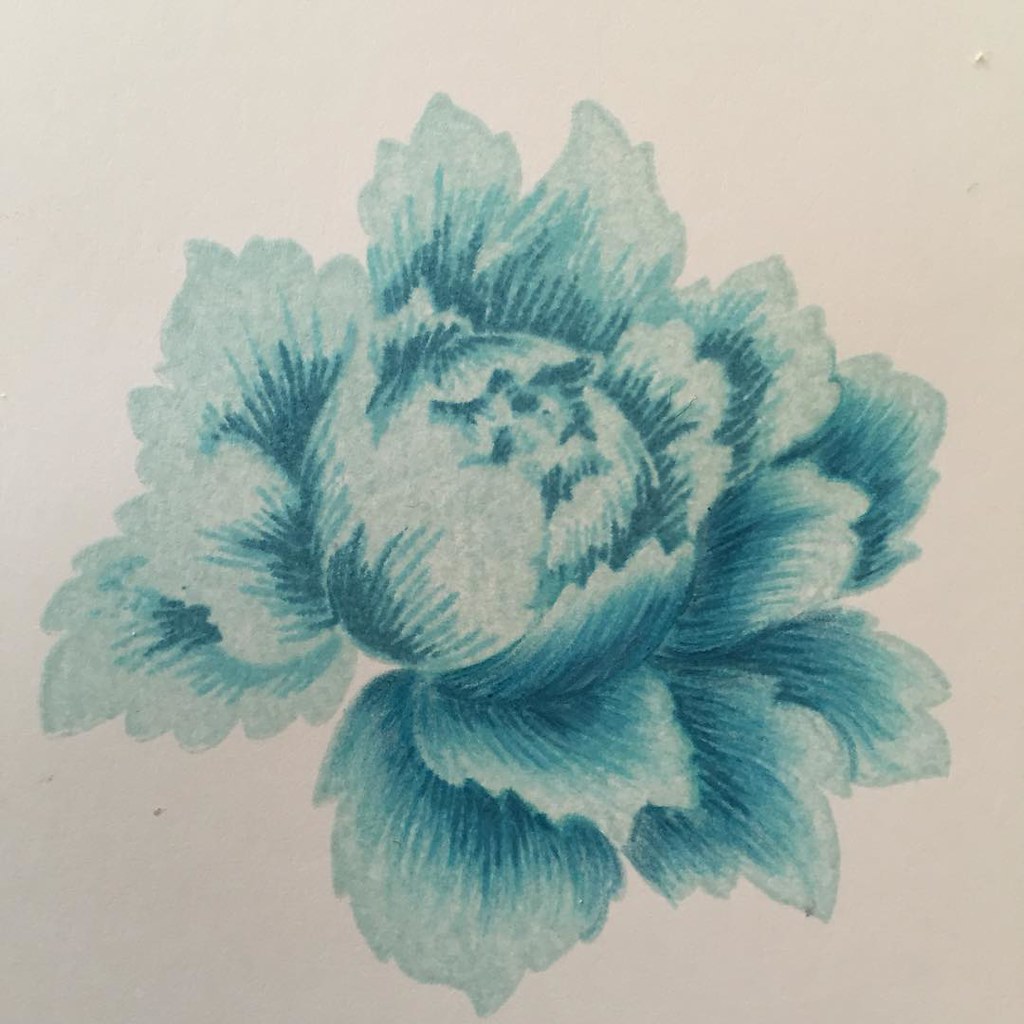This intricate artwork showcases a detailed floral head against a white background. Predominantly shaded in hues of blue, the flower features a mesmerizing gradient, transitioning from darker blues at the center to lighter edges that nearly blend into the white canvas. The flower is depicted with three concentric layers of petals, each petal meticulously drawn to reveal visible veins, lending a lifelike texture to the painting. At the core, the flower's center appears just beginning to open. Notably, the painting employs significant negative space, allowing the background to highlight the flower's form. The overall composition, centered on the canvas, is characterized by an almost circular formation with multiple petals radiating from the orb-like center. This beautiful blend of detailed line work and gradient shading successfully highlights the artistry embedded in the simple, yet striking, flower representation.